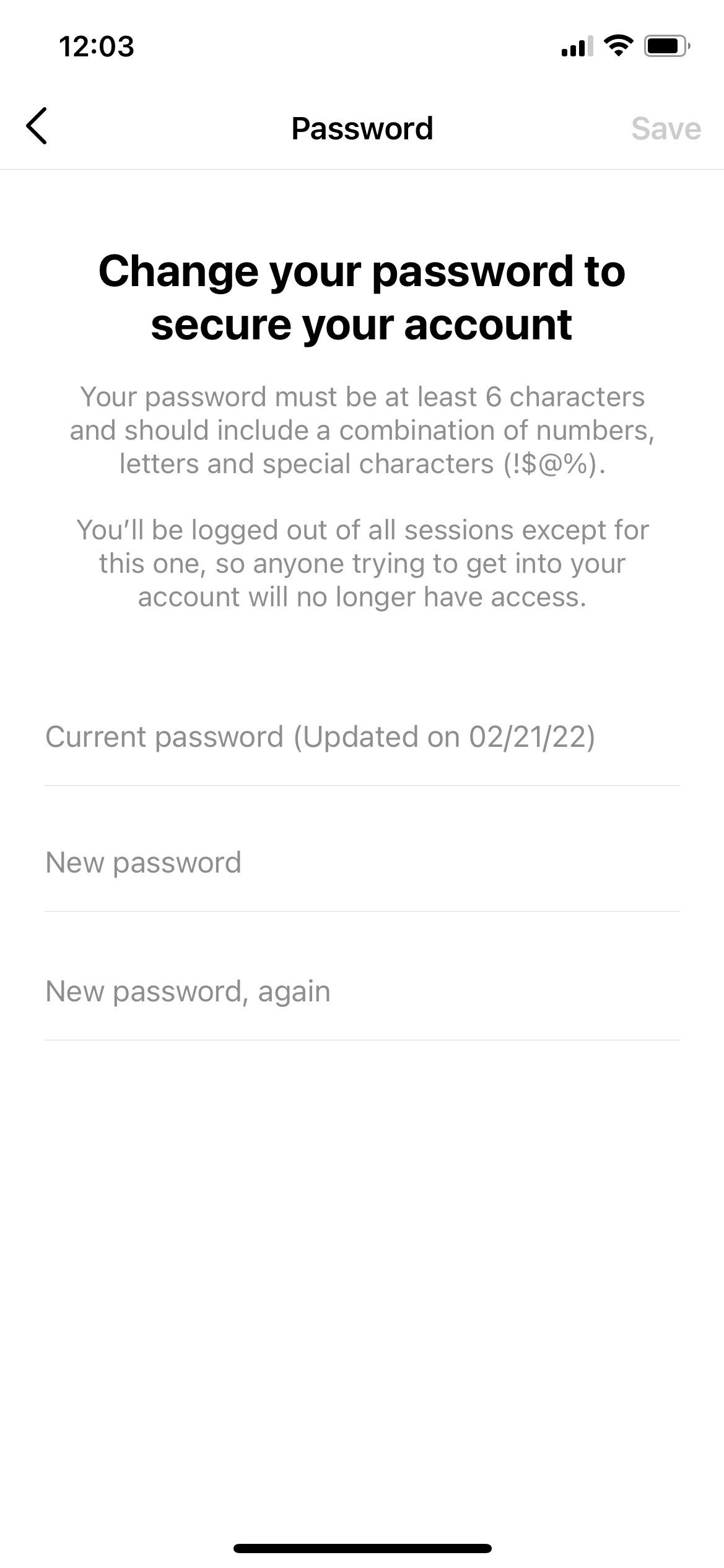The image depicts an iPhone screen displaying an application's password change interface. The iPhone interface elements are visible, such as the swipe bar at the bottom, the time displayed as 12:03 in the top left corner, signal strength with three bars, four bars of Wi-Fi, and roughly 80% battery life. The application's interface shows a back button on the top left and a "Save" button on the top right. In the center, the header reads "Change your password to secure your account." Below, it provides guidelines: the password must be at least six characters long and include a mix of numbers, letters, and special characters (e.g., exclamation point, dollar sign, at symbol, or percentage). 

The notice also informs the user that changing the password will log them out of all sessions except the current one so that unauthorized users will be logged out. The form below the instructions includes fields for the current password (last updated on February 21, 2022), followed by two fields for the new password, requiring the user to enter it twice to confirm it matches.